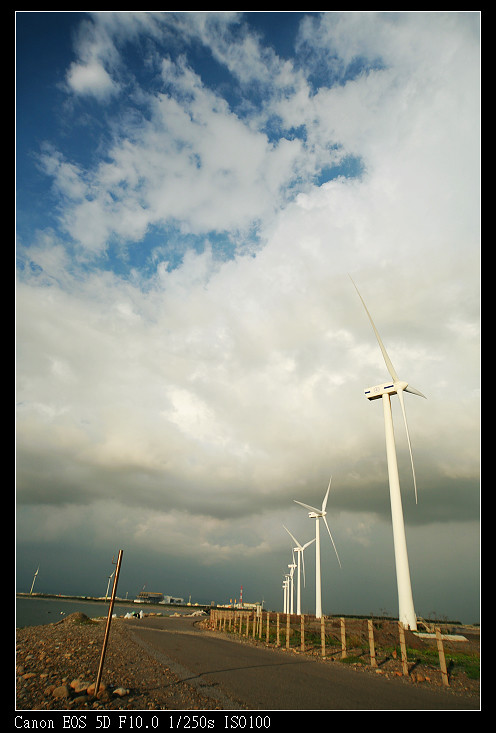This outdoors photo, taken with a Canon EOS 5D (F10.0 1/250s ISO100), captures a dramatic landscape dominated by the sky, which makes up nearly 90% of the image. The sky exhibits a mix of thick white and gray clouds, with hints of blue peeking through the top left corner. The bottom portion of the photograph features a winding road that curves from the bottom right and disappears into the distance, leading to a small building. To the left of the road, there are gravel rocks and a glimpse of the coast with water visible near the buildings. On the right side of the road stands a line of at least six tall, white wind turbines with three blades each. A barely visible thin-wire fence runs to the left of the turbines, blending into the expansive scene. This view is framed by a subtle black border, enhancing the image’s depth and detail.